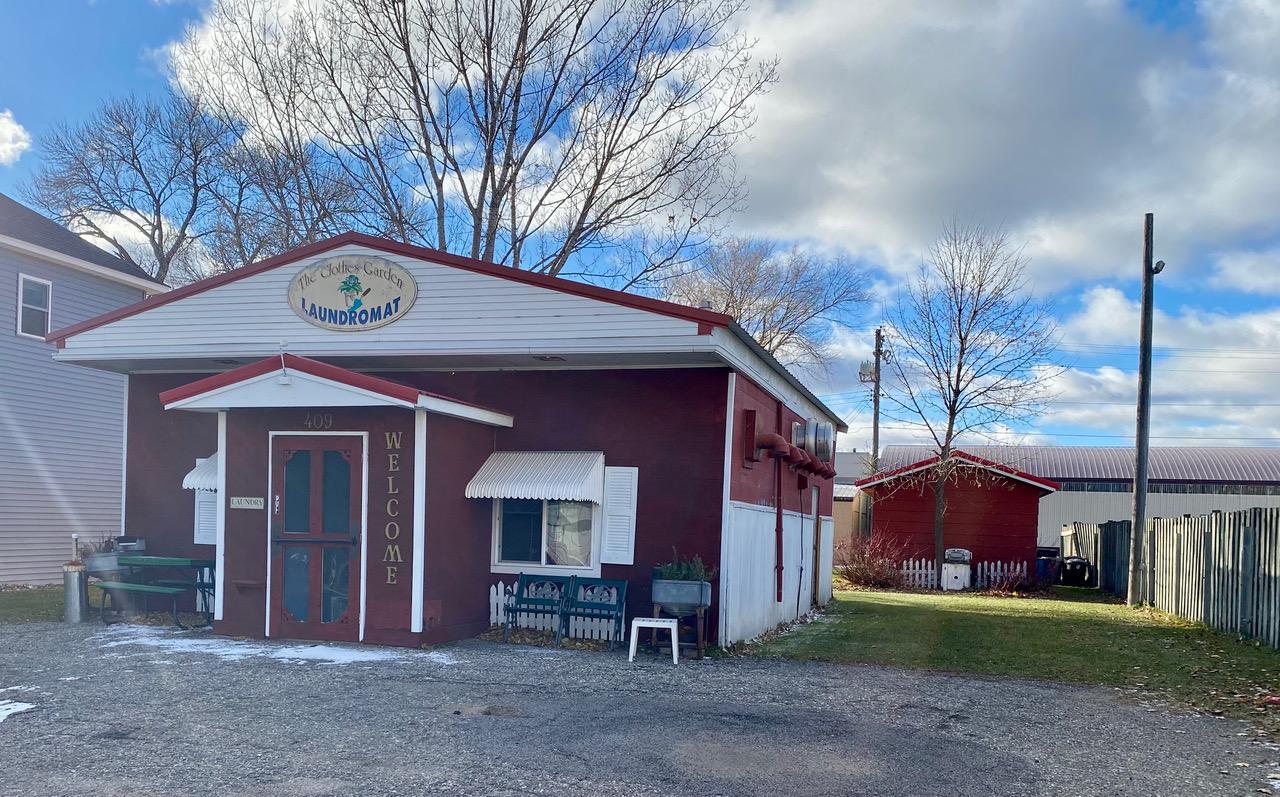In this full-color, square photograph taken outdoors on a partly sunny day, the scene captures a quaint neighborhood laundromat known as The Clothes Garden Laundromat. The sky is a mix of blue and fluffy white clouds, with bare tree branches reaching upward. The focus is the red and white, single-story, ranch-style building. Prominently displayed above the entrance is the laundromat’s sign, featuring an oval-shaped logo with an image of someone doing laundry. The entrance, centered on the flat part of the building, displays the address, 409, along with a welcome sign beside the door. 

The building is bordered by a rustic wooden fence that extends from the lower left corner of the image. A couple of light posts and a power line are also visible. In front of the laundromat, there are white awnings above the windows, a large bench, a picnic table to one side, and remnants of snow on the ground. The background showcases a red shed to the rear and a large home to the left. The natural light and partly sunny conditions create a balanced illumination over the entire scene, highlighting the comfort and community atmosphere of this local laundromat.